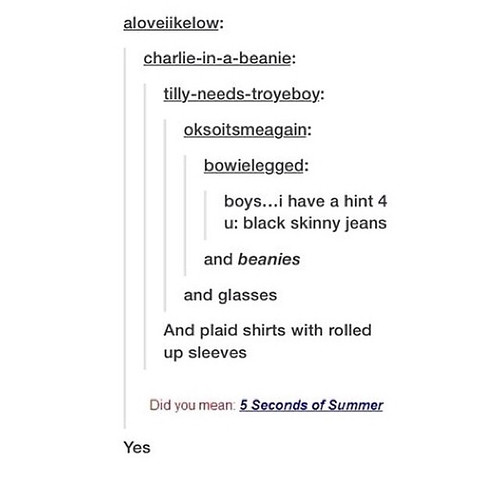The image depicts a black and white graphic with a hierarchical chat-like structure featuring various lines of black text on a white background, resembling a series of text messages or group chat. At the top, it starts with "A love like [our]" and includes a list of names and phrases such as "Charlie - in a beanie," "Tilly - needs Troy boy," and "Bowie legged." 

The central part includes a message saying, "Boys, I have a hint for you," followed by descriptive clues including "black skinny jeans," "beanies," "glasses," and "plaid shirts with rolled up sleeves." Towards the bottom, in red writing, it queries, "Did you mean Five Seconds of Summer?" with an affirming response, "Yes," highlighted in blue as a link. The text collectively hints at a playful guessing game where users identify the described subject, who is ultimately revealed to be the band Five Seconds of Summer.